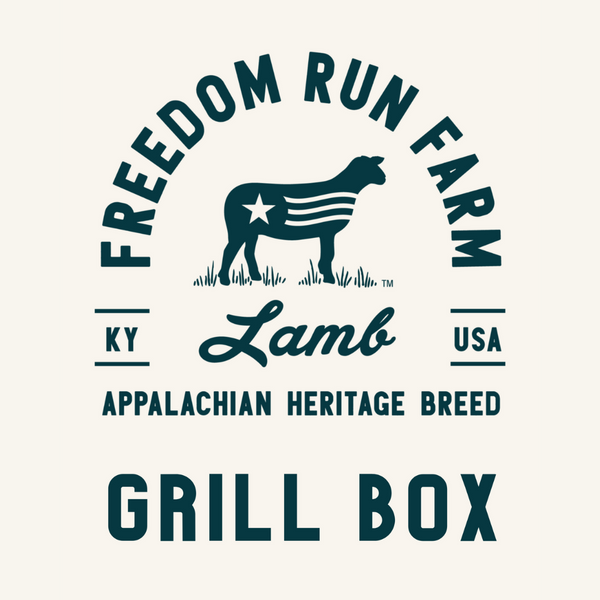The image is a digital graphic featuring a brand label with a simple yet detailed design. It hasa text line at the top formed into an arch shape, reading "Freedom Run Farm" in dark green lettering. Below this arch, there is an artistic depiction of a lamb standing on grass, with its body adorned with a star and three wavy lines. To the left of the lamb is the small text "KY Kentucky USA," and beneath the lamb is the script word "lamb." Further, underneath, it reads "Appalachian Heritage Breed" in all caps, followed by "GRILL BOX." This entire design is in a single deep green color, set against a solid light grayish-greenish background that occupies the majority of the image space. The graphic is simplistic yet striking, primarily employing black, white, and green hues.